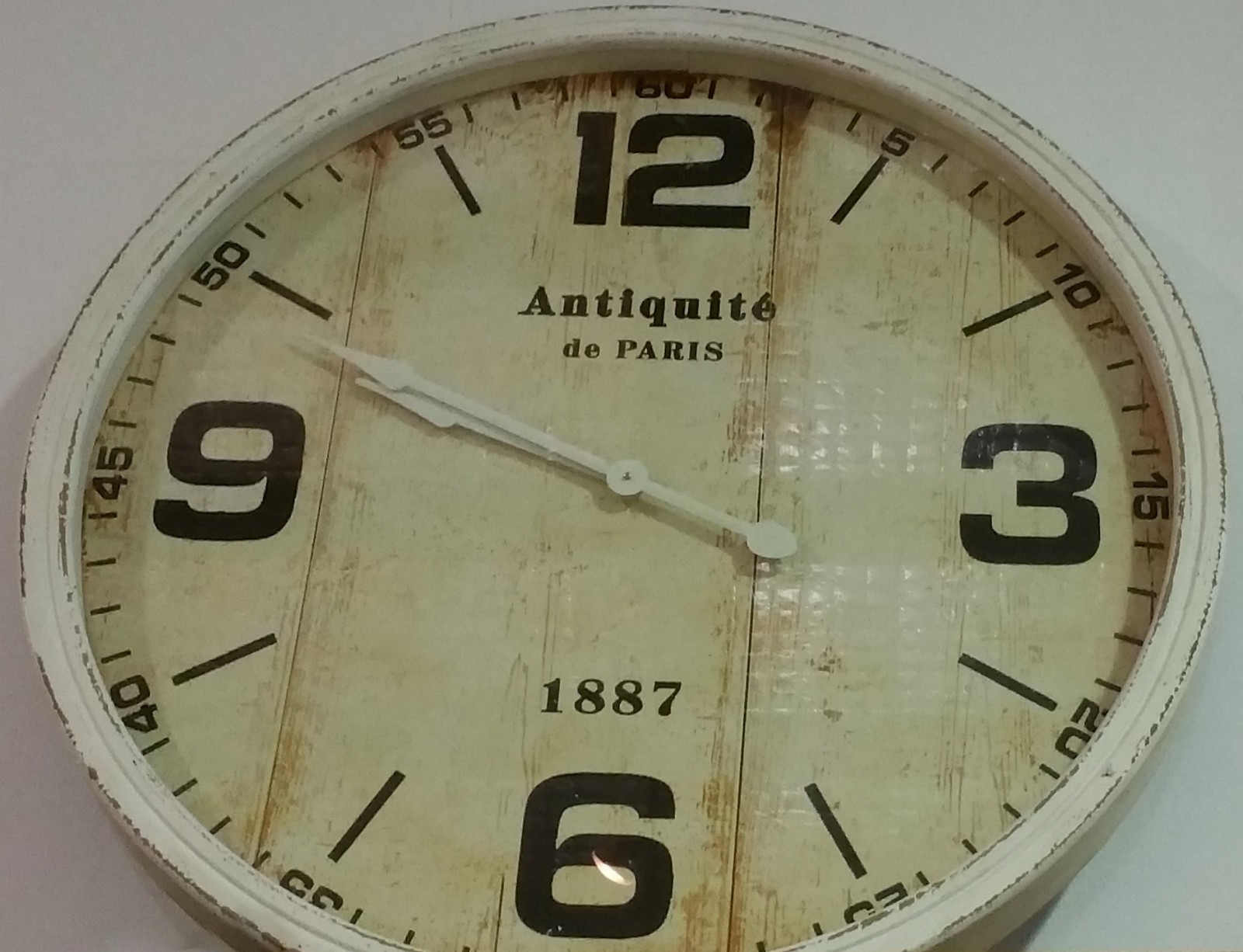The image depicts a rustic, shabby chic style clock with a distinctively antique appeal. The face of the clock appears to be made from white painted boards with visible vertical seams, giving it a worn, distressed look. Surrounding the face is a white ring, which reveals underlying gray or brown tones due to areas of rubbed-off paint, adding to its vintage appearance.

The clock's hour and minute hands are both white, designed with a pointed arrow at one end and a circle at the other. They are positioned just shy of the number 10, indicating the time as approximately 9:48. The numbers on the clock face are in black, with the Arabic numerals for 12, 3, 6, and 9 prominently displayed. The remaining hour markers are represented by black oblique lines. In addition, the minutes are labeled in increments of five, starting from 5 next to the 12 and increasing up to 60 above it.

Above the number 6, the face of the clock features the text "1887," grounding its antique aesthetic. Below the 12, the inscription reads "Antiquité de Paris," with an accented 'E,' suggesting French origins. The overall background of the image is an off-white, likely a wall, further highlighting the clock's old-fashioned charm. Despite its weathered look, the hands of the clock remain in good condition, contrasting with the overall distressed finish of the piece.